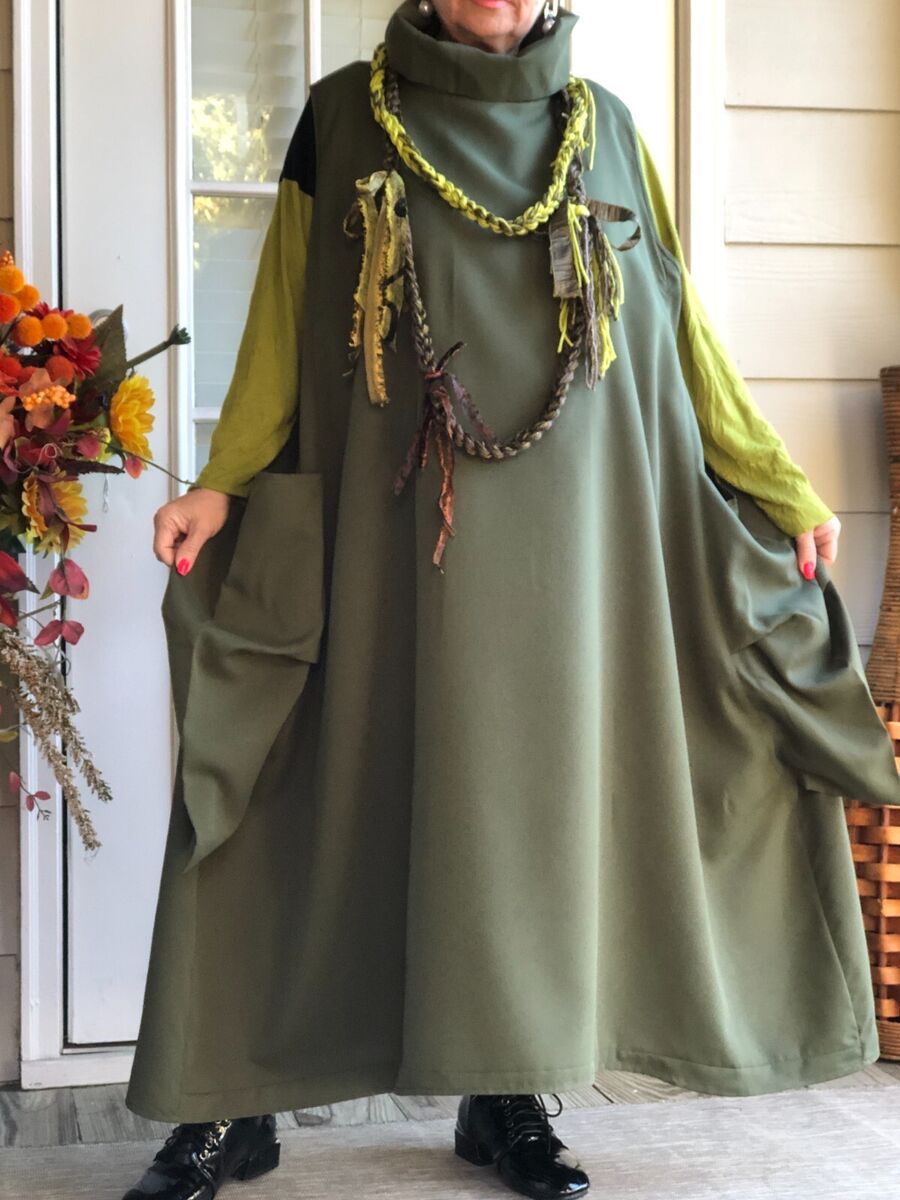A professionally photographed color image features an older woman standing outside on a porch. Her face is cut off, revealing only her mouth and chin adorned with pink lipstick. She wears a long olive green caftan with light green crepe material draping over her hands, which are polished with bright pink nail polish. The caftan has large pockets that she holds, creating an A-line shape. Around her neck, she sports intricately beaded fabric necklaces, one with green and gray woven cords, draping almost to her waist. Her outfit is completed with shiny black lace-up boots featuring a modest one-inch heel. To her right, a wicker basket stands near the center of the image, while hints of flowers peek in from the left. Soft, professional lighting enhances the entire scene, highlighting the details of her attire and the surrounding porch.